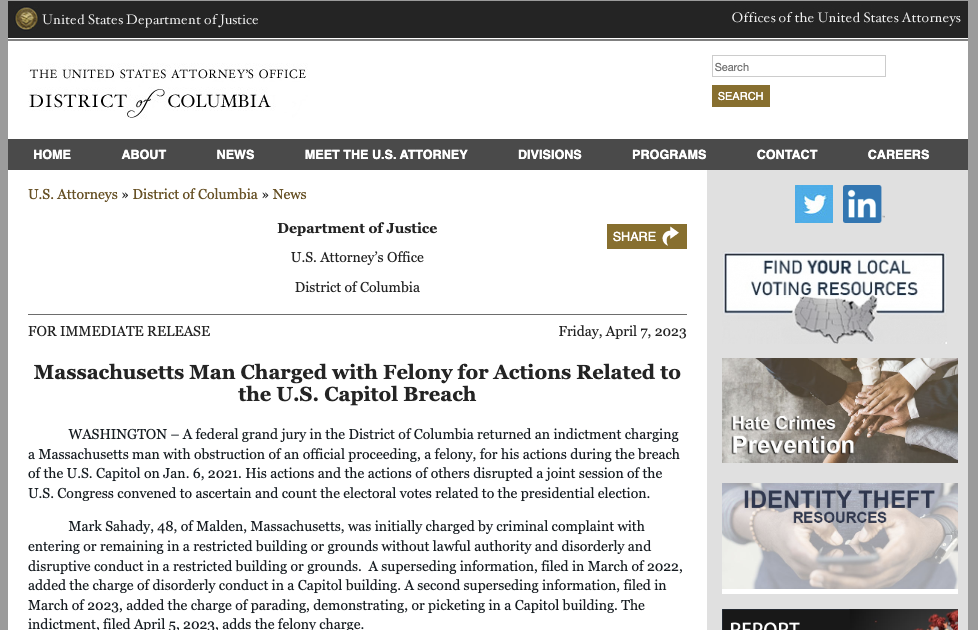The image depicts a webpage from the United States Department of Justice, specifically the Offices of the United States Attorneys, with a gray outline and a prominent black header. The header features the DOJ emblem to the left and links including "Home," "About," "News," "Meet the U.S. Attorney," "Divisions," "Programs," "Contact," and "Careers."

Beneath this header is a white background area designated for the United States Attorney's Office for the District of Columbia. At the top of this section, there is a search box accompanied by a brown search button. The left side of this white background includes a section labeled "U.S. Attorney's District of Columbia News," further detailing that it is associated with the Department of Justice and the District of Columbia.

Further down, under "For Immediate Release," it is dated Friday, April 7, 2023, and details a news release: A Massachusetts man has been charged with obstruction of an official proceeding, a felony, related to the January 6, 2021, breach of the U.S. Capitol. The suspect, Mark Sahadi of Malden, Massachusetts, initially faced charges for unlawfully entering and disrupting a restricted building. Subsequent charges included disorderly conduct in a Capitol building in March 2022, and parading in a Capitol building in March 2023, culminating in the recent felony indictment filed on April 5, 2023.

On the right side of the page, there is a blue box providing links and information about local voting resources, hate crimes prevention, and identity theft resources.